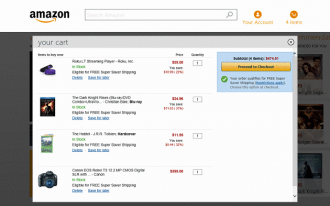A low-resolution screenshot from the Amazon website showcases a user's shopping cart filled with four items. The cart window is prominently displayed on top of another, now greyed-out, Amazon browsing window. At the very top of the image, the Amazon logo and search box are visible, alongside an account icon and an indicator showing four items in the cart.

The highlighted "Your Cart" section includes a settings button and a "Proceed to Checkout" button. Below these, there is a list viewing the added items, each accompanied by a small, blurred image to the left, a brief description, the price, and quantity. While the specific items are not clear, due to the low resolution, one appears to be a camera and another a video game.

In essence, the screenshot captures a user’s prepared Amazon shopping cart, ready for checkout, set against the familiar Amazon interface backdrop.